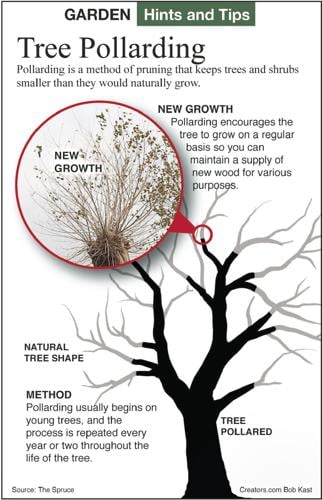This infographic, titled "Garden Hints and Tips," focuses on the practice of tree pollarding. The title "Hints and Tips" is displayed prominently in white lettering against a green background. The infographic features an illustration of a wiry tree with a dark trunk and lighter gray branches. A key callout highlights a specific upper branch, labeled as "New Growth," accompanied by a detailed zoomed-in view of this area. This close-up shows new stems and leaves, emphasizing the effects of pollarding.

The text explains that pollarding is a pruning method for maintaining trees and shrubs at a smaller size than their natural growth. Pollarding promotes regular new growth, ensuring a continuous supply of new wood for various uses. The description clarifies that pollarding typically starts with young trees and is a recurrent process, performed every one to two years throughout the tree's life.

Additional notes on the infographic include terms like "Natural Tree Shape," "Method," and "Tree Pollard," sourced from The Spruce. Smaller, less readable text is present, but the main focus remains on illustrating and explaining the practical benefits of pollarding.